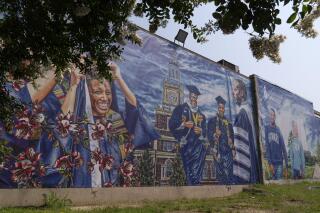The image depicts a large mural covering the entire side of a three to four-story building, free of windows on this wall. The mural, painted in predominantly blue, white, and brown hues with some skin tones, illustrates a graduation ceremony. Several graduates, dressed in blue and white caps and gowns, are standing in front of what seems to be a significant college or university building with a backdrop of blue sky. To the right side of the mural, there are figures in blue and green sweatshirts, possibly branded with the college name, although the distance makes it hard to decipher. Surrounding the mural, green grass stretches along the base of the building, and tree branches with dark green leaves drape into the upper corners of the scene, adding a natural frame. A small brown half-wall is visible at the bottom of the image, enhancing the mural's depth and realism. The mural's intricate details and expansive dimensions express a vibrant and lively tribute to the academic milestone.